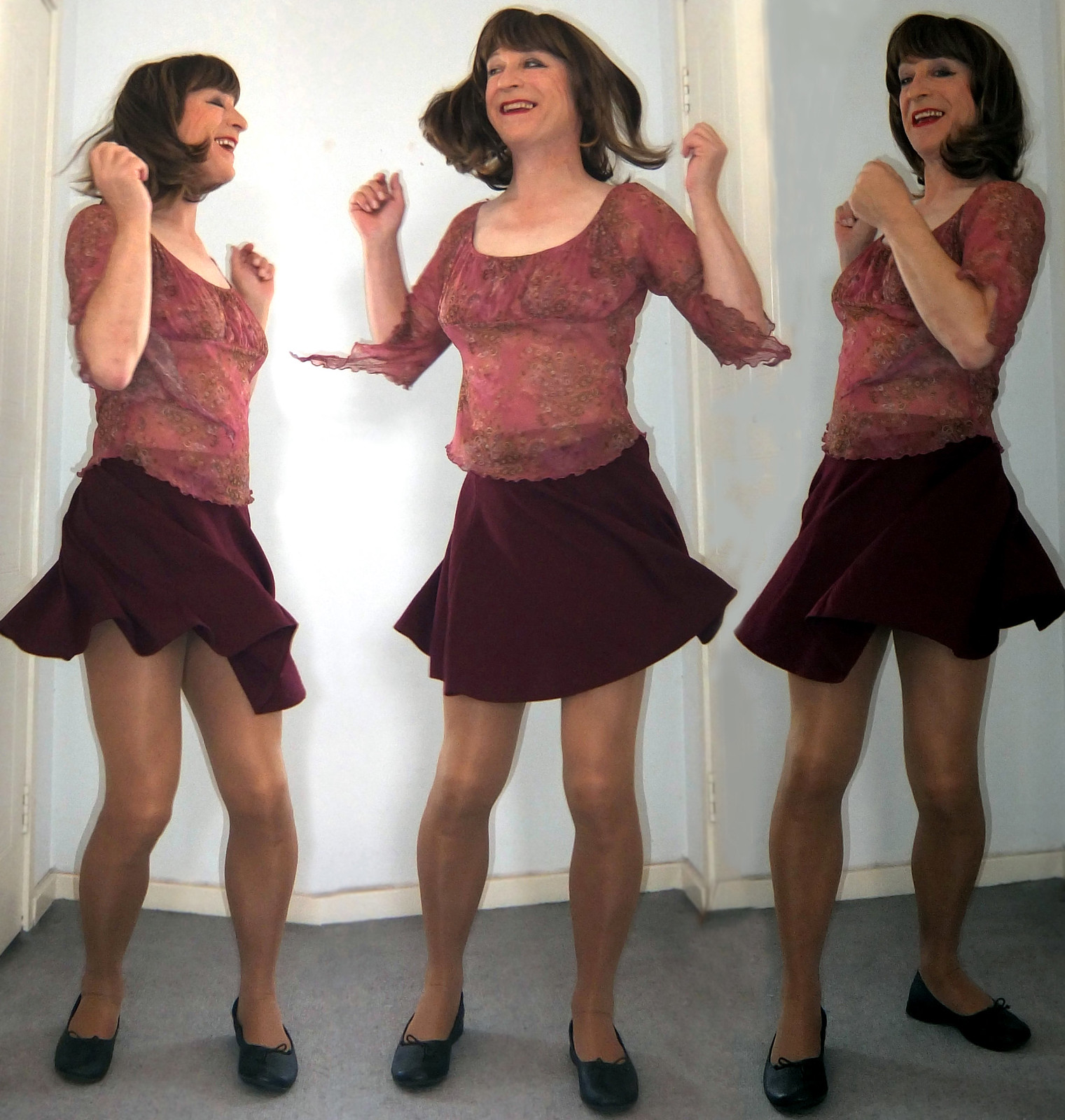The photograph is an indoor collage featuring three images of a jubilant woman, possibly a man dressed as a woman or a transgender woman, captured dancing. Her dark brown bob with a fringe frames her face adorned with red lipstick, with her hair playfully flying out as she moves. Each image shows her smiling broadly, exuding joy.

She wears a sheer, floral, lacy top in shades of burgundy and pink, with elbow-length, flared sleeves, complemented by a deep burgundy, flared miniskirt. Her outfit also includes American tan tights and black ballet flats. The woman's arms are raised in each image, emphasizing her dancing movements. Her body is posed differently in each shot: facing and interacting with her other images, with her skirt swirling and her entire figure animated against a plain white background on a gray floor. The overall impression captures her exuberance and the dynamic nature of her dance.